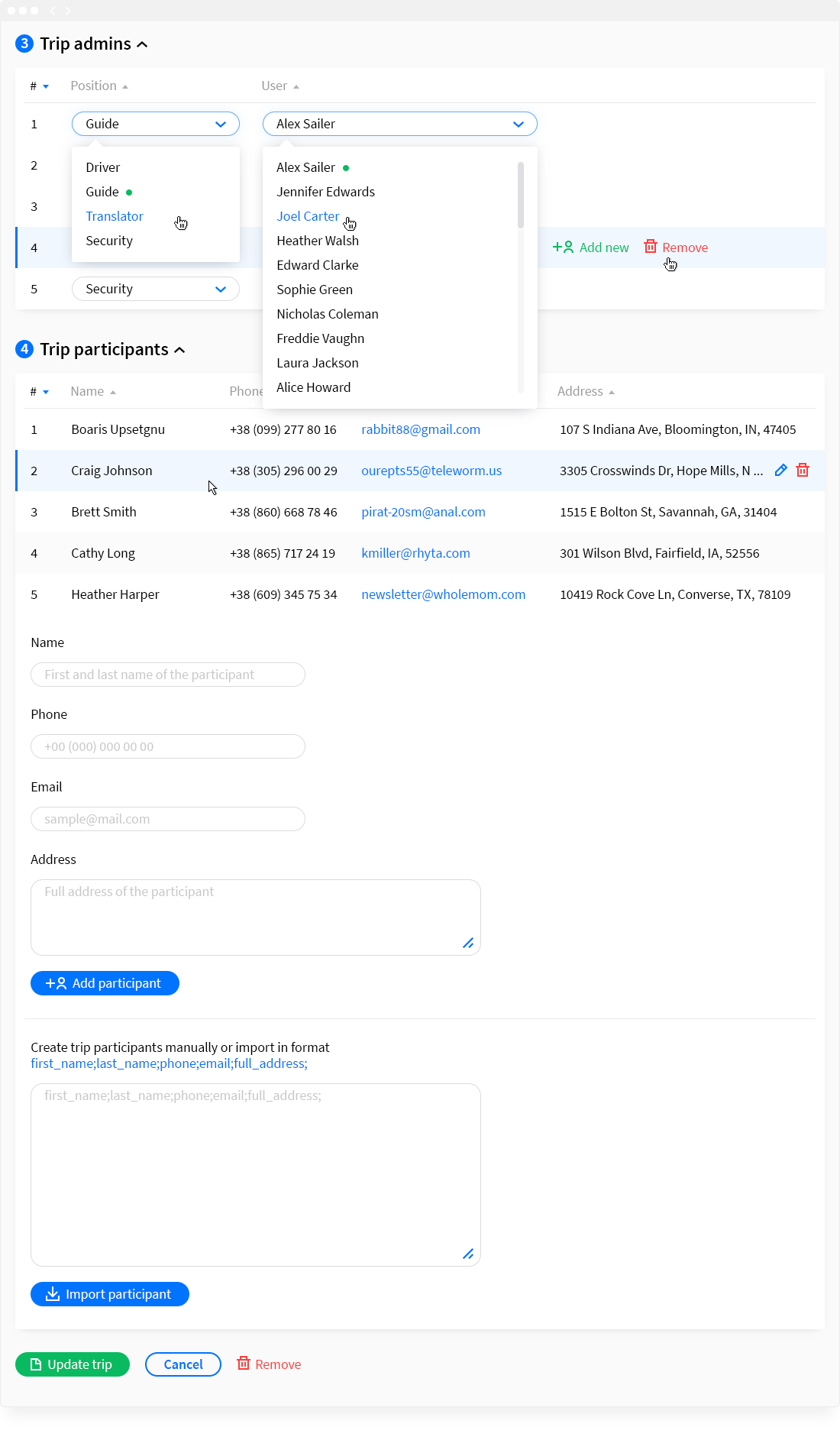A screenshot of a data entry form, heavily reduced in size to the point of being nearly unreadable. The form appears to be a captured segment of a larger web interface, featuring a pale gray bar across the top with illegible text. Beneath the bar, the primary background is predominantly white. 

At the top of the form, a blue circle with the number '3' inside precedes the label "Trip Admins," followed by a caret symbol. Below this header is a grid with three columns containing multiple rows of data.

- **First Column:** Numbered items from 1 to 5.
- **Second Column:** Titled "Position," featuring a dropdown box currently displaying "guide." The dropdown options include "Driver," "Guide," "Translator," and "Security."
- **Third Column:** Titled "User," with the user "Alex Saylor" currently selected. The dropdown list contains additional user names: Jennifer Edwards, Joel Carter, Heather Walsh, Edward Clark, Sophie Green, Nicholas Coleman, Freddie Vaughn, Laura Jackson, and Alice Howard.

The form is designed for trip administration, presumably allowing users to assign different roles to various individuals listed.